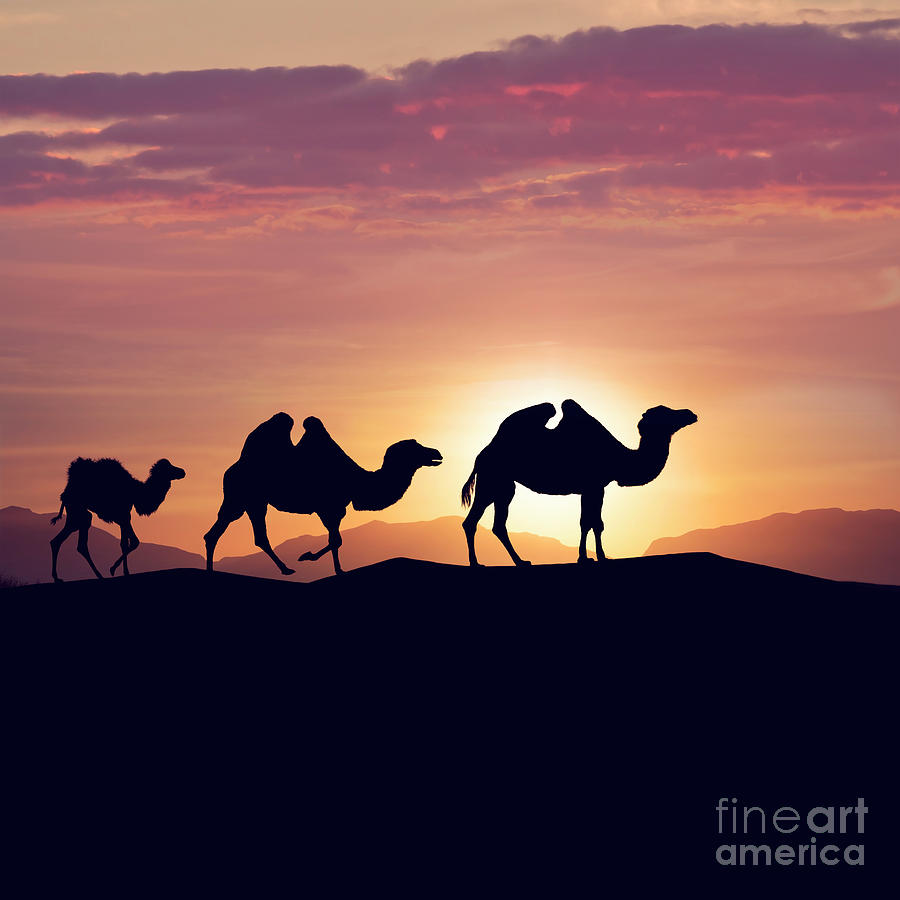In this captivating image, three camels stroll across a desert hill at sunset, their figures rendered in dark, striking silhouettes. The two larger camels and one smaller camel form a stunning procession against a backdrop of vivid colors: deep purples, fiery oranges, and golden yellows grace the sky, scattered with wisps of clouds. The sun, just peeking above the low-lying mountains on the horizon, casts a soft glow, partially eclipsed by the rightmost camel's silhouette. There are no reins or signs of ownership on these camels, lending an air of wild, untamed beauty to the scene. The serene and majestic atmosphere, coupled with the fine details, such as the shadowed camels and the ethereal desert landscape, evokes a sense of tranquil solitude. At the lower right-hand corner of the image, the words "Fine Art America" subtly mark its origin.